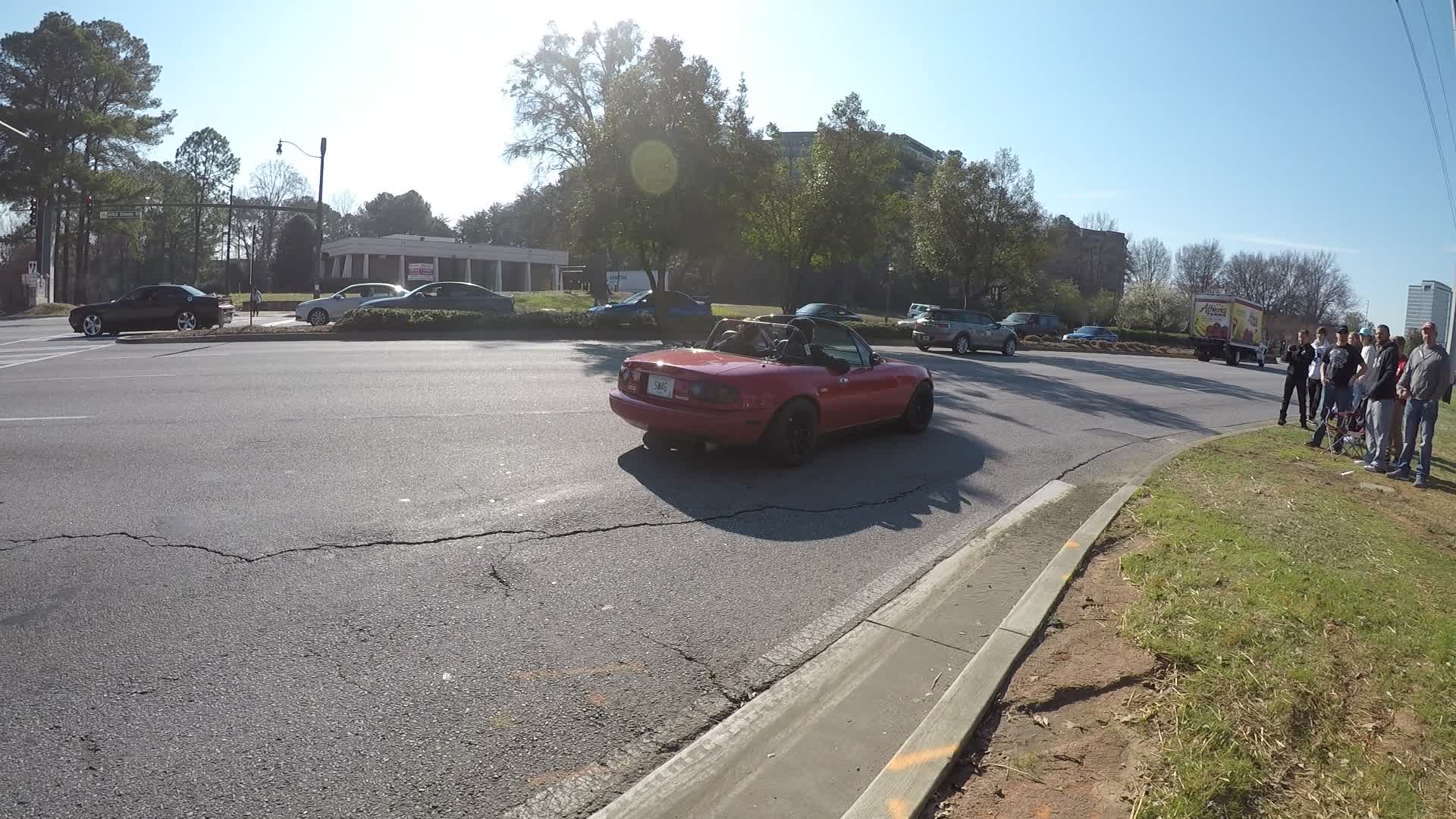This vibrant street scene captures a dynamic city environment during the day. At the focal point is a red convertible Miata, roof down, as it navigates the street, possibly in a spirited turn. This lively Miata, carrying a couple of passengers, appears to be part of a car show or meet, which is suggested by the presence of a crowd gathered along the sidewalk on the right side of the road. The street is divided by a grassy median adorned with trees, and more spectators can be seen on the opposite side, eagerly observing the scene. The backdrop features a mix of urban elements, including an apartment building in the back right, several brick structures varying from one to three stories, and a stoplight positioned on the back left. Traffic is visible, with cars and a large truck waiting at a stoplight on the opposite lanes. The blue sky and sunny conditions enhance the lively atmosphere of this city event.